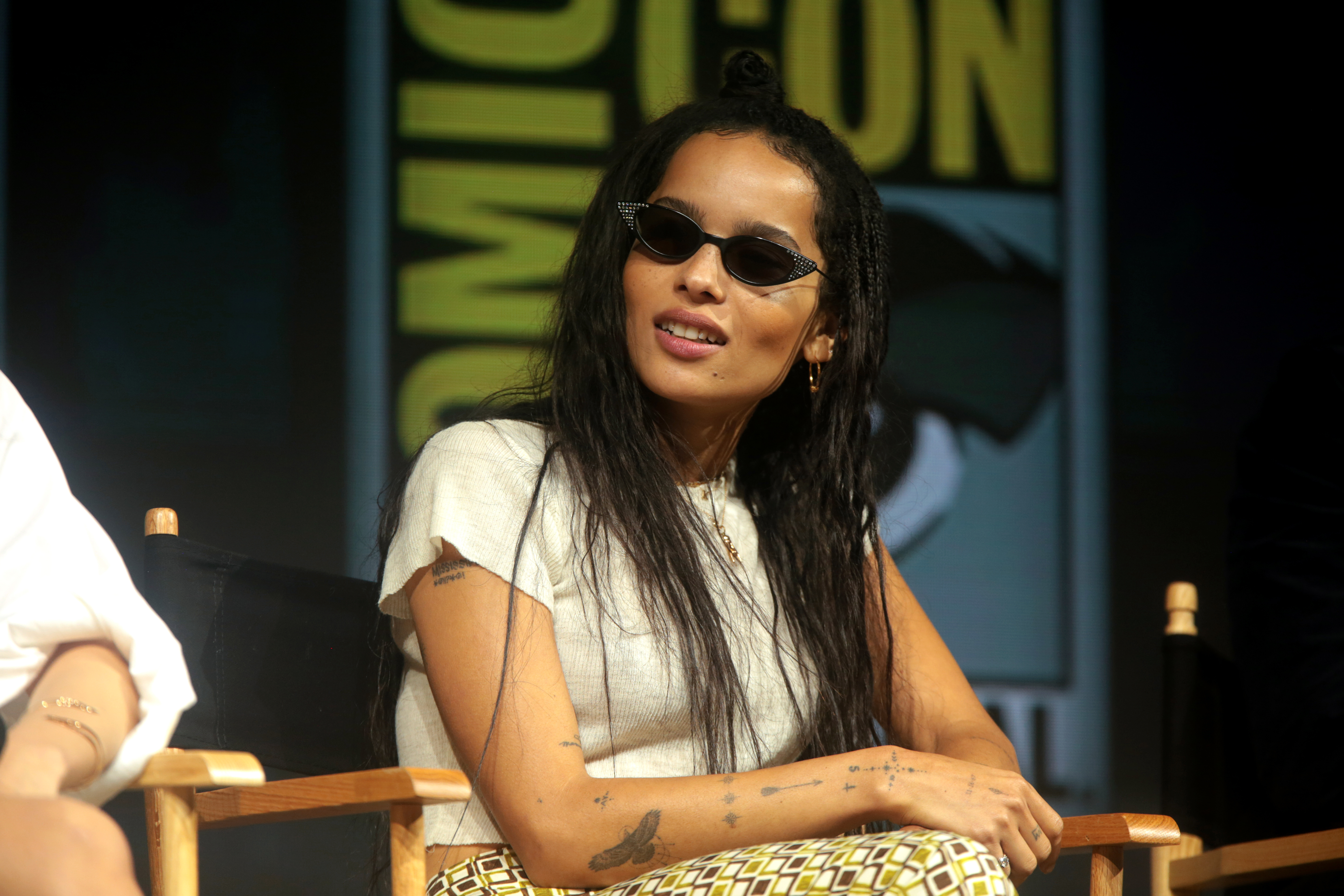In this image from Comic-Con, Zoe Kravitz is seated centrally in a dimly lit room, occupying a wooden director's chair with a black fabric back. She is wearing distinctive black cat-eye sunglasses embellished with gems. Her attire consists of a cropped cream-colored ribbed shirt and yellow pants adorned with a pattern of alternating brown and tan squares. Her long, brown hair cascades almost to her stomach. Notably, her right arm displays a variety of tattoos, including an eagle, an arrow, and several other designs. Although the image is slightly blurred, a Comic-Con logo can be discerned in the background. To her right is another chair of similar design, and we can see the arm and knee of another woman seated there, dressed in a white shirt. The overall setting appears to be indoors, likely during an interview or panel discussion.